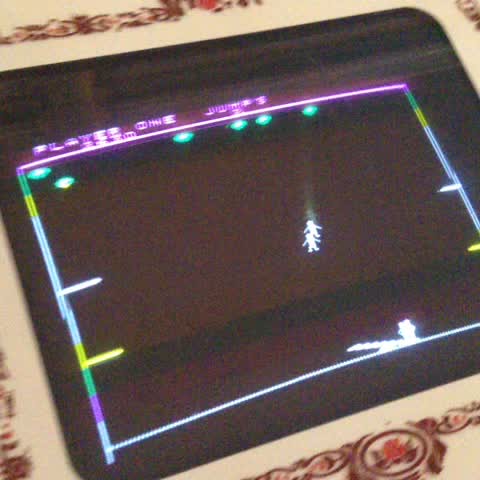This image showcases an extremely vintage video game displayed on a rudimentary, early video monitor. The screen exhibits a basic, heavily pixelated display with minimal detail, characteristic of early digital graphics. The setup features profiles of participants, each positioned on opposite sides with goals clearly marked. The background of the screen is black, with lighter colored elements in white or various hues standing out prominently.

At the top of the screen, distorted and slightly out-of-focus names are visible, likely indicating player names or scores. To the left of the screen, there are diamond or oval shapes that may represent footballs or another game-related item, adding a touch of thematic context. Cream-colored bezels adorned with a floral pattern frame the screen, further emphasizing the vintage aesthetic of this early gaming console. The display also includes minimal data and information, exemplifying the simplistic yet pioneering spirit of gaming in its nascent stage.